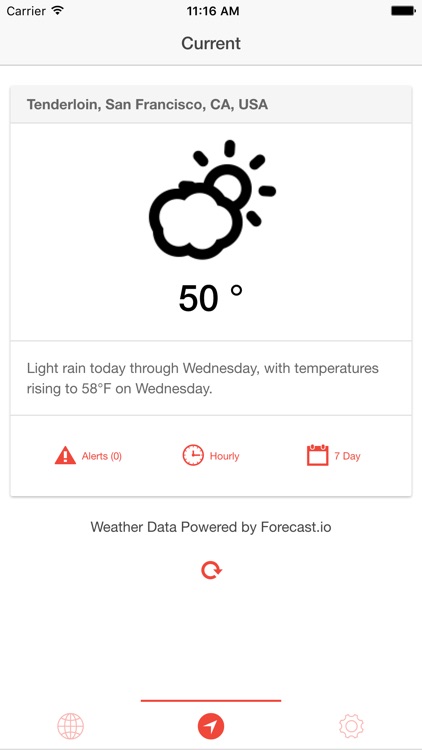A detailed weather report for the Tenderloin neighborhood of San Francisco, California, USA, at 11:16 AM: The temperature is currently 50°F under partly cloudy skies with intermittent sunshine. Light rain is expected to persist today through Wednesday, with temperatures forecasted to rise to 58°F by midweek. The weather data, provided by forecast.io, indicates no current alerts. The display includes various icons such as a refresh symbol, a globe, an arrow within a circle, a settings wheel, and a notable red line, while a fully charged battery ensures uninterrupted updates.